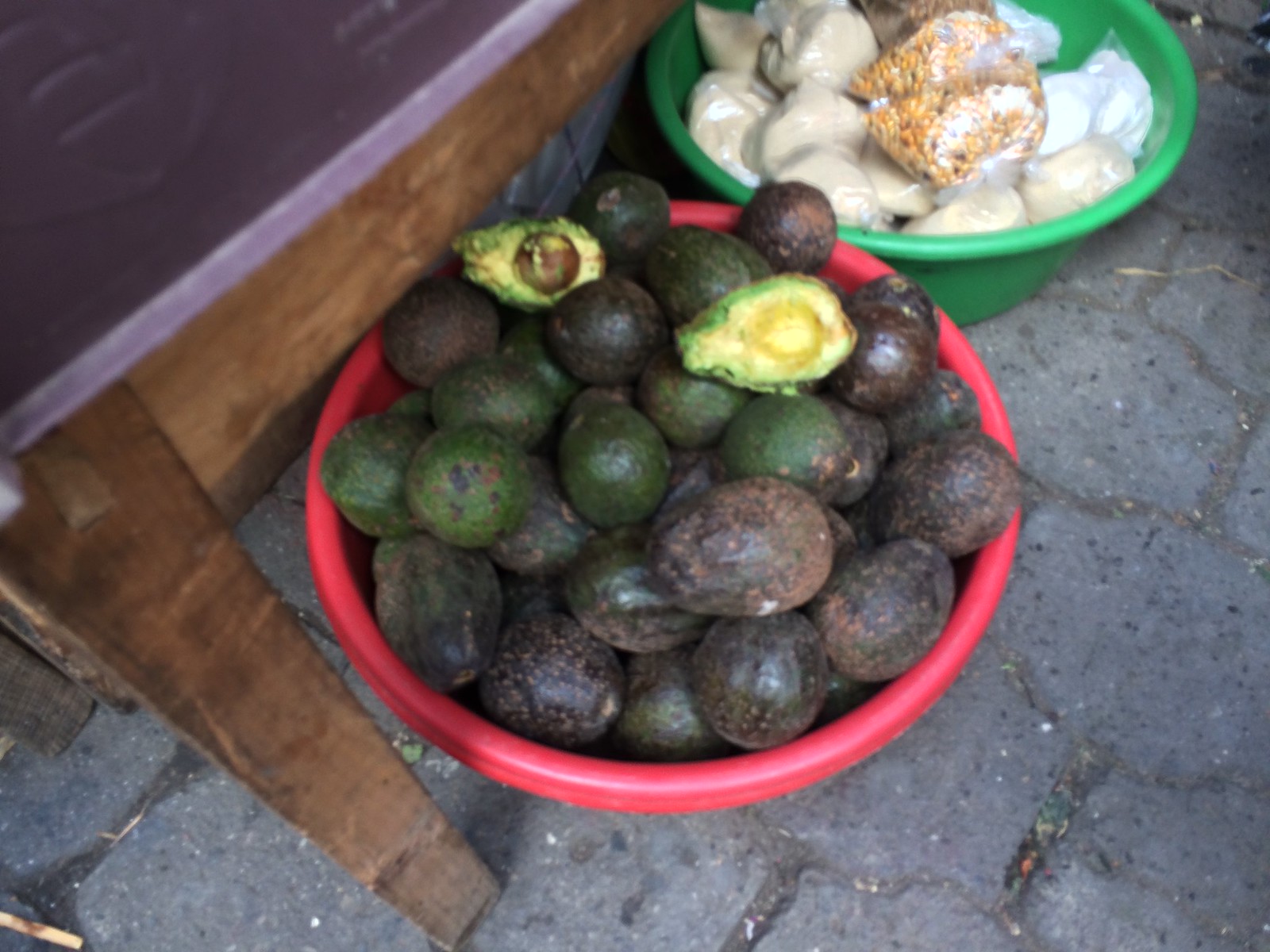In an outdoor setting with an older, gray, hexagonal or pentagonal cobblestone ground, there are two buckets at the foreground. The red bucket is filled to the brim with avocados of varying colors - from dark green to brown with some light beige spots. One avocado is halved, displaying its seed and flesh. Next to it stands a green bucket containing what seems to be chopped durian, with a plastic bag of brown seeds on top. Additionally, the green bucket holds several plastic bags, one with white contents, and others with yellow, orange, and brown items. The scene suggests an aged area in need of cleaning, with vivid contrasts between the fresh and overripe produce.